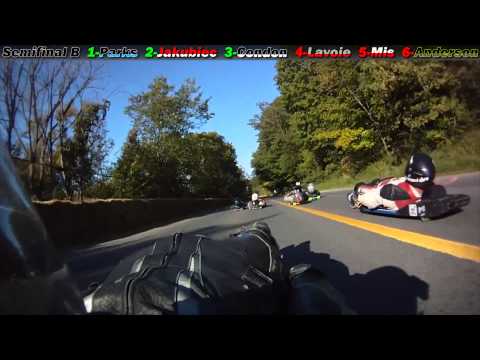The photograph captures an exhilarating luge race from a first-person perspective. The scene features participants lying on full-body luge boards, all wearing helmets for safety. The road they are racing down is asphalt with a prominent yellow stripe running down the middle, navigating through a picturesque outdoor setting with tall, thick green trees flanking both sides. The sky overhead is clear and blue, enhancing the vibrancy of the scene.

In terms of attire, the racers have distinct uniforms: the racer to the right wears a white and red outfit with a black helmet, while another participant in the top left corner sports a black leather outfit, casting a shadow to his right. At the top of the image, visible text indicates the competitive nature of the event, reading "Semi-Final B" followed by the names and rankings of the racers, from 1 to 6: Parks, Jacooby, Condon, LaVoie, Mia, and Anderson. The overall atmosphere is charged with the thrill of speed and competition.